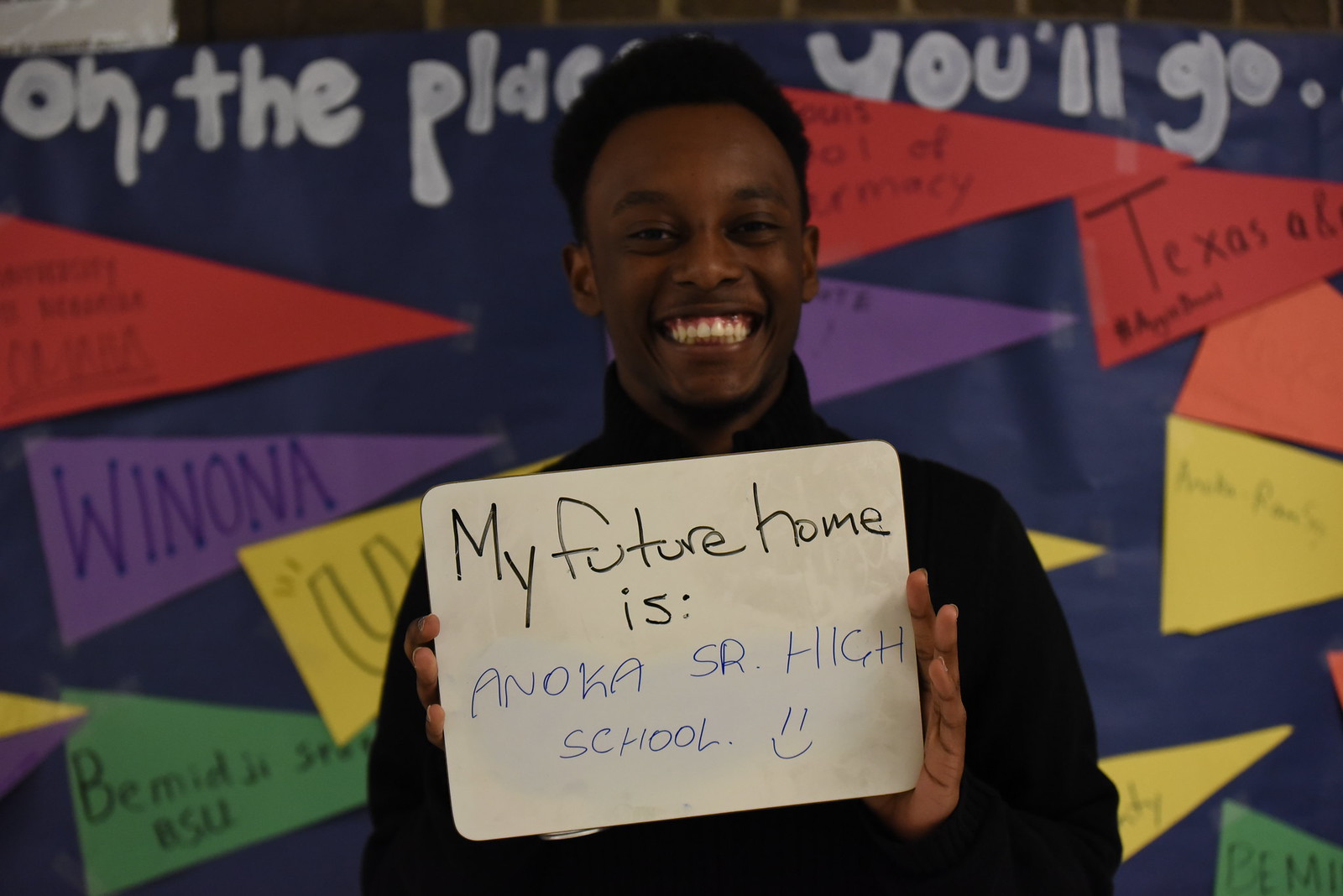The photograph shows a young black man with short hair and a beaming smile, dressed in a black long-sleeve shirt, holding a small white rectangular sign with curved corners. The sign, written in black Sharpie, reads "My future home is Anoka Senior High School" with a cheerful smiley face at the end, where the eyes are two extended lines and the mouth is a letter 'C'. In the background, a large cardboard banner features the phrase "Oh, the places you'll go" in white lettering. Surrounding the banner are triangular flags in red, orange, purple, green, and yellow. These flags bear the names of various colleges such as Winona and Texas A&M, though some are too fuzzy to read clearly. The vibrant display of school spirit and future aspirations suggests this photo was taken during an event celebrating the young man's transition to Anoka Senior High School.